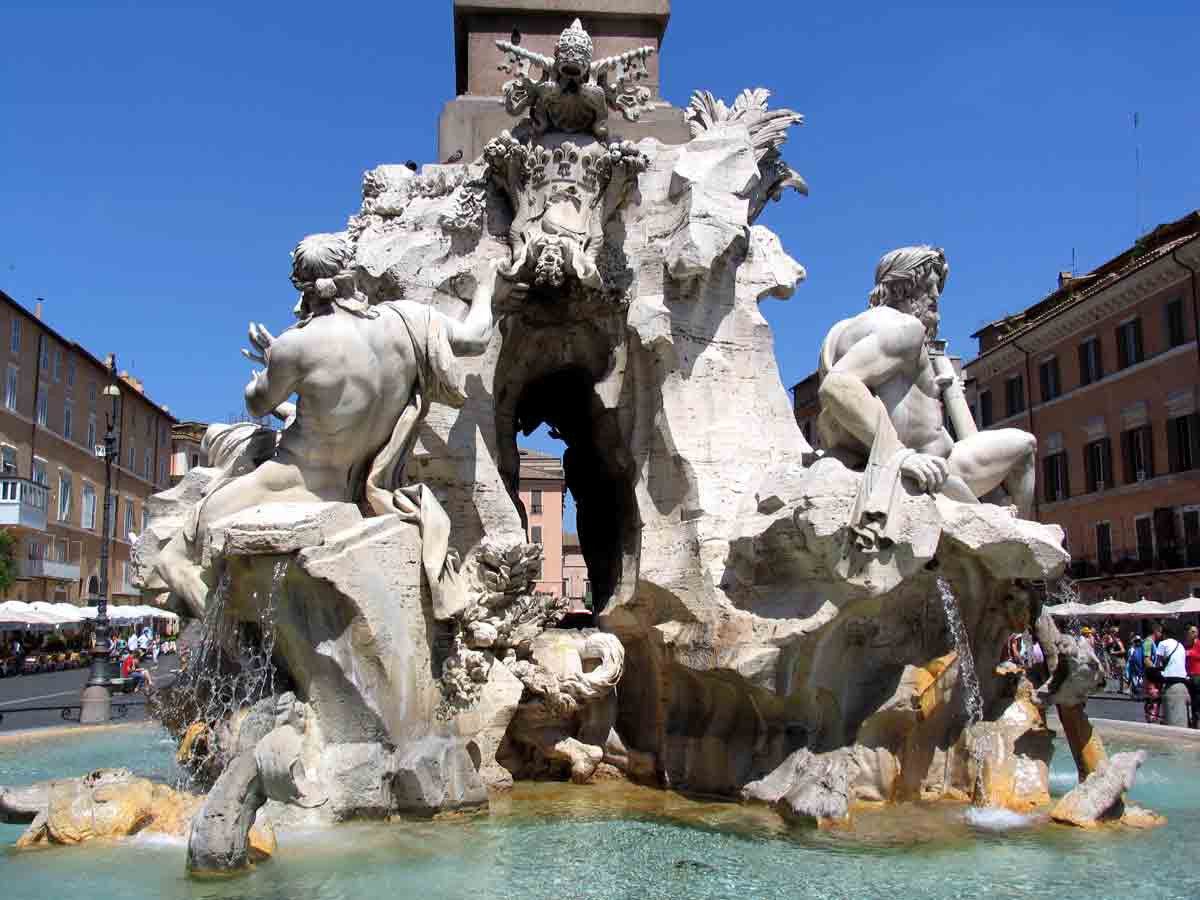The photograph captures a large, ornate fountain situated in a likely European city square, framed by a vibrant, cloudless blue sky. The focal point of the image is an intricate white stone statue rising from the fountain's clear, slightly greenish water. The statue features various figures, including at least two male deities in classical poses, with one gazing upwards toward a mysterious creature perched atop an elaborate arch. The fountain's base is shallow, and its central design includes a hole through which a red brick building in the background is visible. Flanking the fountain are bustling sidewalks populated with pedestrians and approximated by sidewalks cafes, indicated by umbrellas in front of multi-story buildings with a distinct orangish-pink hue. This detailed and lively scene captures the essence of an old-world European urban landscape.